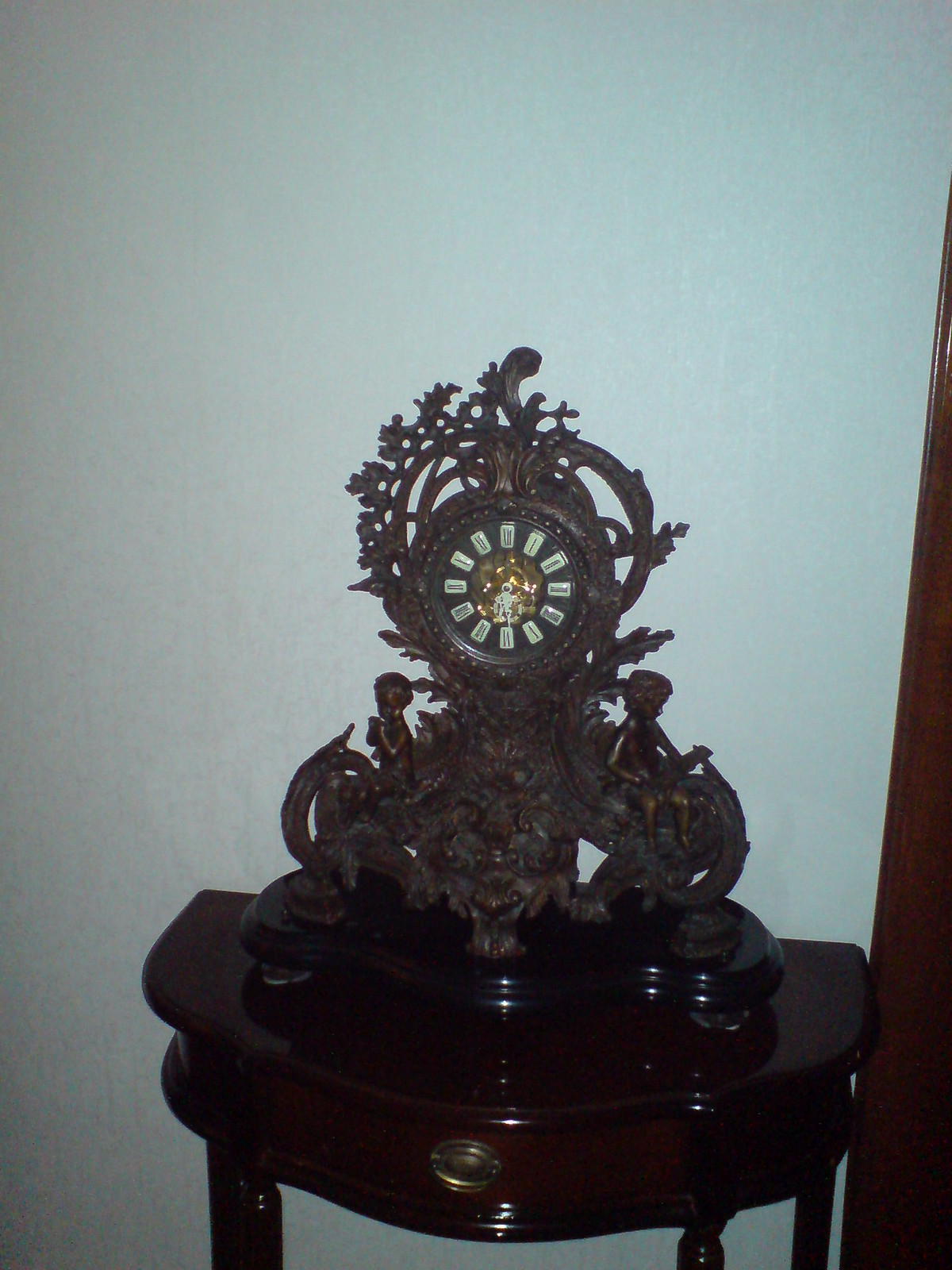The image depicts an intricately designed clock. At the forefront, there are multiple legs supporting the clock, providing a sense of stability and grandeur to the cobblestone setting. This large structure features detailed carvings, including threads at the back that add an element of sophistication. The clock is adorned with a central lion’s face, exuding a majestic and classic aura. Surrounding the lion's face is a hawk motif, blending seamlessly into the design. The clock face showcases Roman numerals from one to twelve, with each number impressively highlighted in black text on white squares. Encircling the middle metal portion—which exudes a regal golden hue—are elaborate carvings of lion-like designs etched into the wood. The clock hands are white and sharply pointed, standing out against the dark, elegant backdrop. The entire piece is bathed in a gentle light, enhancing its timeless and refined appearance.